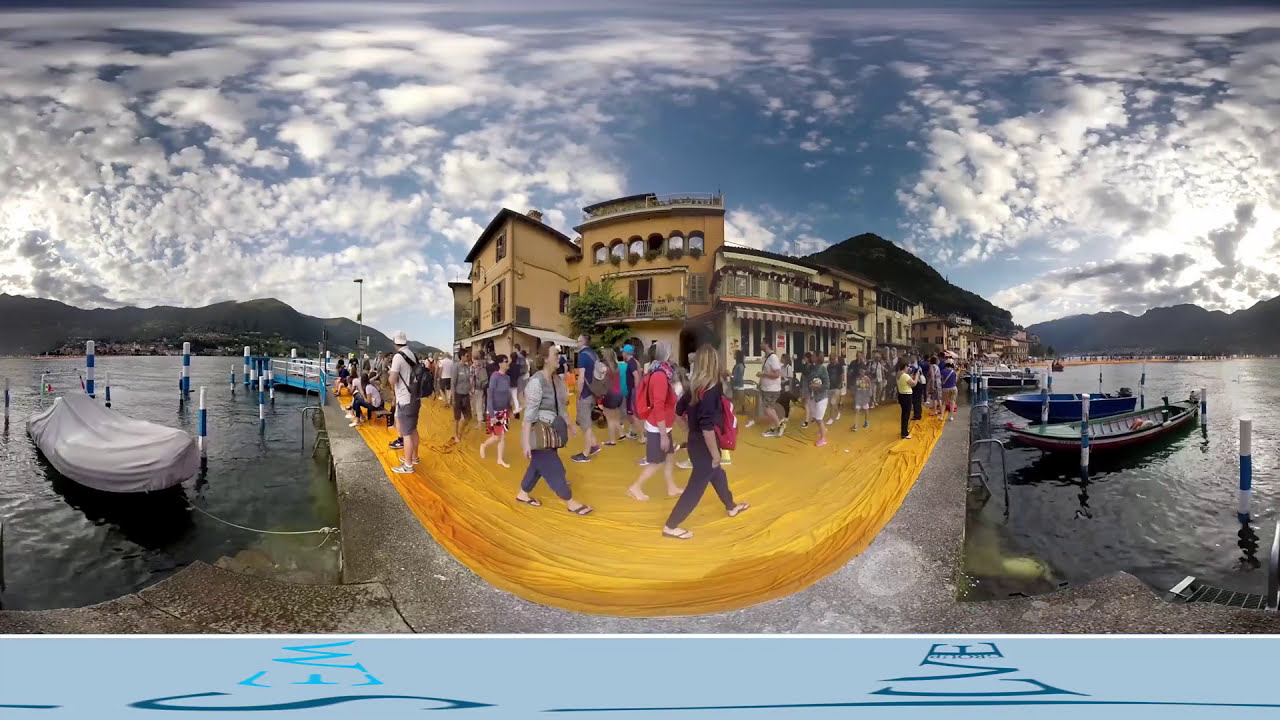This detailed photographic image, taken with a wide-angle lens, captures a bustling outdoor scene during a warm daytime at what appears to be a popular tourist attraction. The wide-angle view causes the sidewalk and the adjacent buildings to curve into a gentle U-shape. This unique perspective shows people strolling along a yellow-tinted sidewalk, surrounded by a picturesque setting where a body of water lies on both sides of the street. Boats, including one covered with a tarp and others tied to blue and white moorings, are anchored nearby. 

Among the crowd, several figures stand out: a woman in a black shirt and pants with black sandals leads the group, followed by another woman carrying a purse, wearing gray attire and also donning black sandals. Trailing behind, a barefoot woman in shorts and a gray shirt walks along. Additionally, a man stands at the edge of the street, gazing at the water while dressed in a white baseball cap, white shirt, and carrying a black backpack. Other notable individuals include a man in a black jack shirt and blue pants, another with goggles, shorts, and a similar shirt, and a woman in a yellow shirt and black pants.

Surrounding this lively scene are several notable buildings. To the right, a small boat is anchored by the street. The backdrop features a mix of older, European-style brown and white buildings, some with colorful awnings, reaching about two to three stories high. An unusual textured yellow material covers parts of the ground. A pier extends into the water, inviting further exploration. A tree grows beside one of these buildings, adding to the appeal of the scene.

Framing the entire scene are majestic mountains that stretch across the image, with a sky filled with white puffy clouds accentuating the blue sky, although the day is slightly cloudy. The sun starts to cast long shadows, hinting its setting behind the mountain range. In the background, there are letters that appear to spell "LVE" in the bottom right-hand corner of the photograph. Overall, the image encapsulates the charm and vibrancy of a waterfront promenade with its lively atmosphere and scenic beauty.